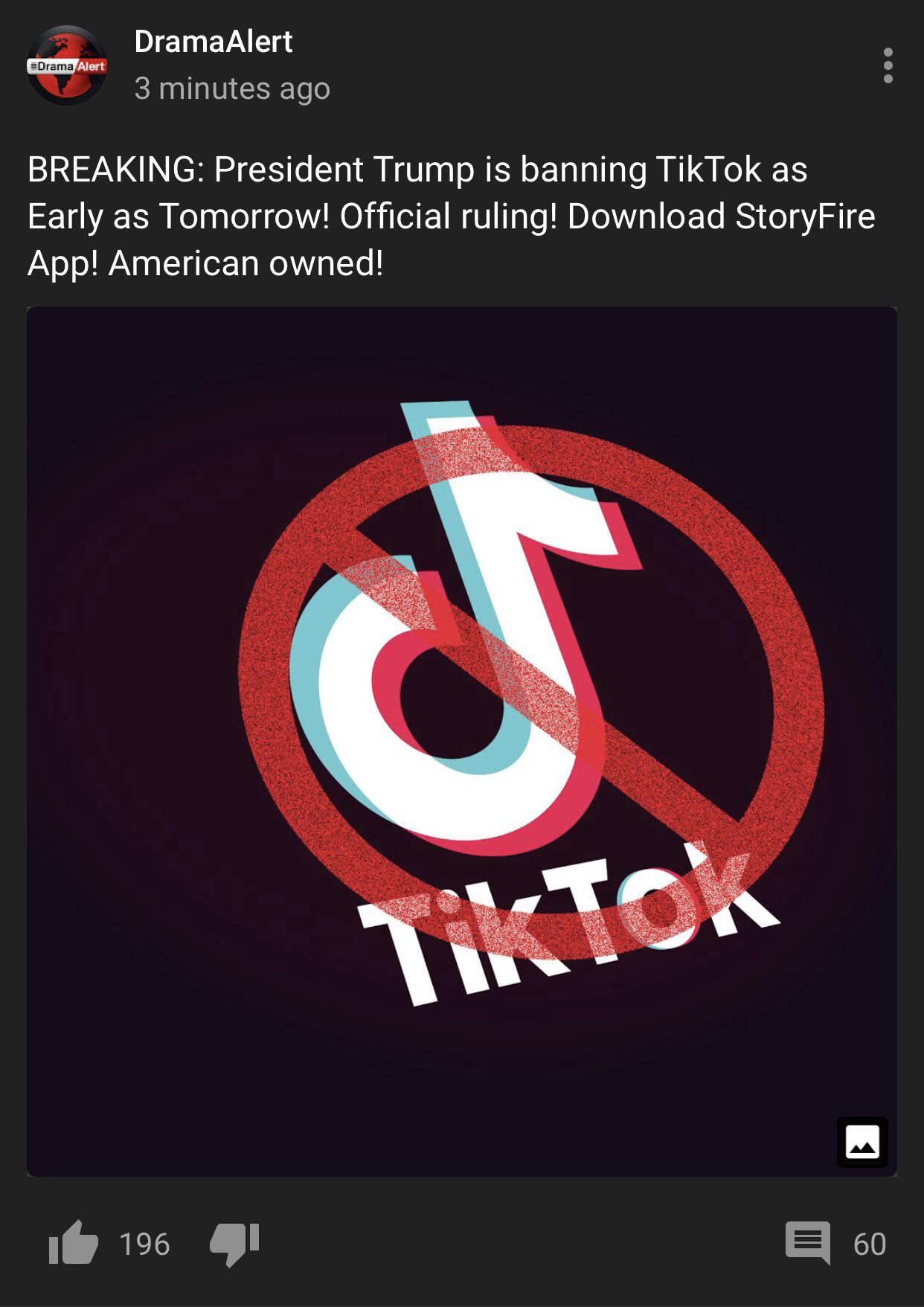The image is a vertical rectangular screenshot of a social media post on a black background. The top left corner features the avatar of DramaAlert, followed by the username "DramaAlert" to the right. The post's headline, written in all caps, reads: "BREAKING: President Trump is banning TikTok as early as tomorrow. Official ruling. Download StoryFire app. American owned." Below this text, there is a large image of the TikTok logo, overlaid with a red prohibition symbol, signifying a ban. At the bottom of the post, there are 196 thumbs-up reactions, 0 thumbs-down reactions, and an icon indicating 60 comments in the bottom right corner.